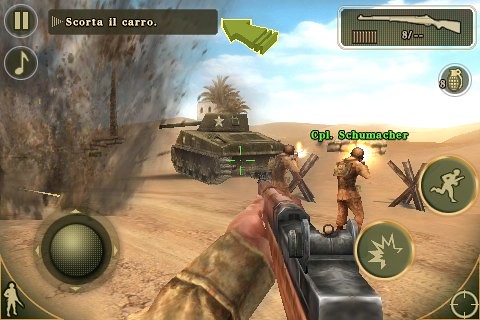Screenshot from a mobile game resembling an early "Call of Duty" or "Battlefield" title, reminiscent of PlayStation 1 graphics. The game appears to be played on an iPhone, given the presence of on-screen controls. A virtual analog stick is visible, used for player movement, along with various action buttons activated by the user's other thumb. The in-game scene depicts the player firing at a tank in a desert-themed level, evocative of older console game environments.